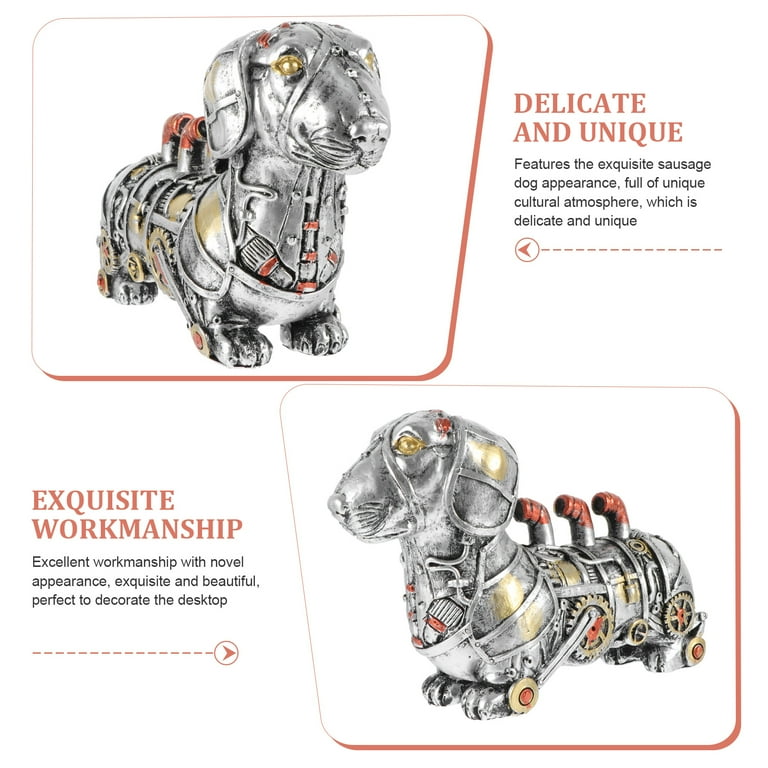This square advertisement features a white background with two images of a steampunk-inspired metal dachshund sculpture, each placed within a faint orange frame with a white background and slightly curved corners, tilted opposite to one another. The top left image presents the dachshund from a forward angle, while the bottom right image shows it from a left-facing angle. This silver sculpture, accented with yellow and orange parts, is adorned with small gears, cogs, tubes, and three distinctive smokestack-like pipes on its back, lending it a unique mechanical appearance. Beside the upper sculpture, an orange title reads "delicate and unique," followed by black text stating, “features the exquisite sausage dog appearance full of unique cultural atmosphere, which is delicate and unique.” Adjacent to the lower sculpture, another orange title reads "exquisite workmanship," with black text underneath describing, “excellent workmanship with novel appearance, exquisite and beautiful, perfect to decorate the desktop.”